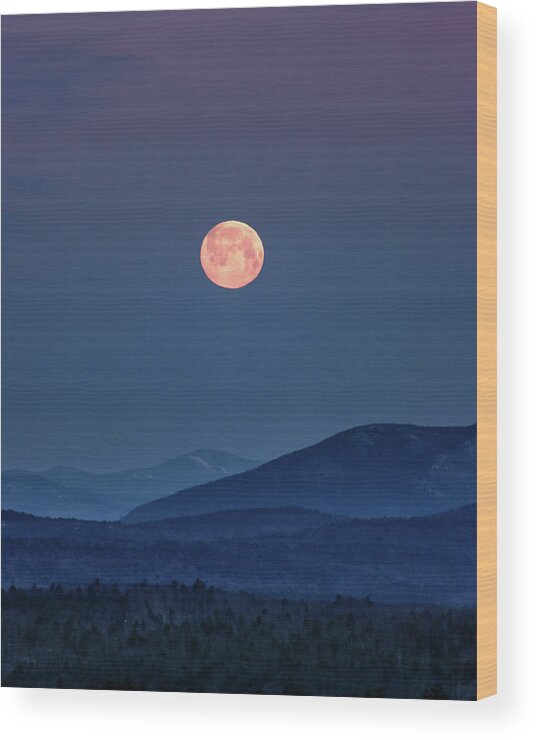The image is a detailed painting on a thick, possibly wooden canvas, depicting a serene night scene in a desert or sparsely populated area. Dominating the dark blue sky at the center is a very large, highly detailed full moon with a pinkish-white hue, adding a dramatic focal point. Below the moon, several layers of blue-gray mountain ranges are visible, creating a sense of depth. In the foreground, there are dark, shadowed sections of ground interspersed with small bushes and green trees that evoke a sparse forest covering about the bottom fifth of the painting. The use of dark, bluish hues throughout the sky and mountains enhances the nocturnal atmosphere.